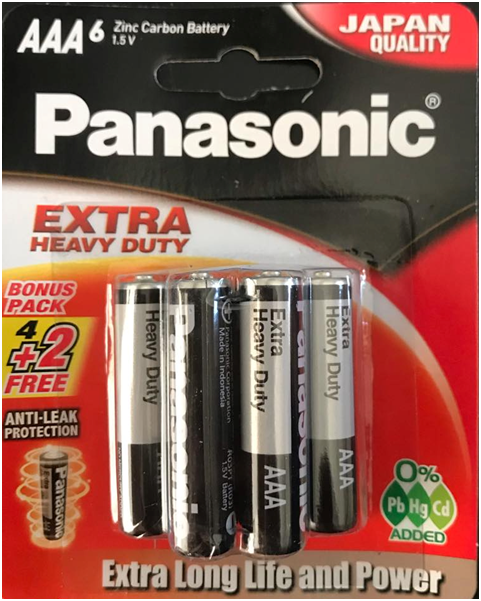This image features a Panasonic AAA Zinc Carbon Battery package, labeled prominently with the Panasonic brand. The package contains a bonus pack of six batteries, which includes four batteries plus an additional two free batteries. These batteries are rated at 1.5 volts and are described as "Extra Heavy-Duty," indicating they are designed to provide high power and long-lasting performance for your devices.

The packaging highlights the inclusion of "anti-leak protection," which ensures the batteries won't leak and potentially damage electronic devices. The environmental benefits are also noted, boasting 0% added mercury and 0% added cadmium, making them a safer option for both users and the planet. The batteries come with a quality assurance label citing "Japan Quality," which is indicative of high manufacturing standards and reliability.

Additionally, the packaging emphasizes "extra long life and power," suggesting these batteries are engineered to outperform standard batteries in terms of longevity and efficiency. It's important to note that these are not rechargeable batteries, but their quality and durability are highly regarded. The package showcases "Zinc Carbon 1.5V" batteries, indicating they are a dependable choice for various high-drain applications.